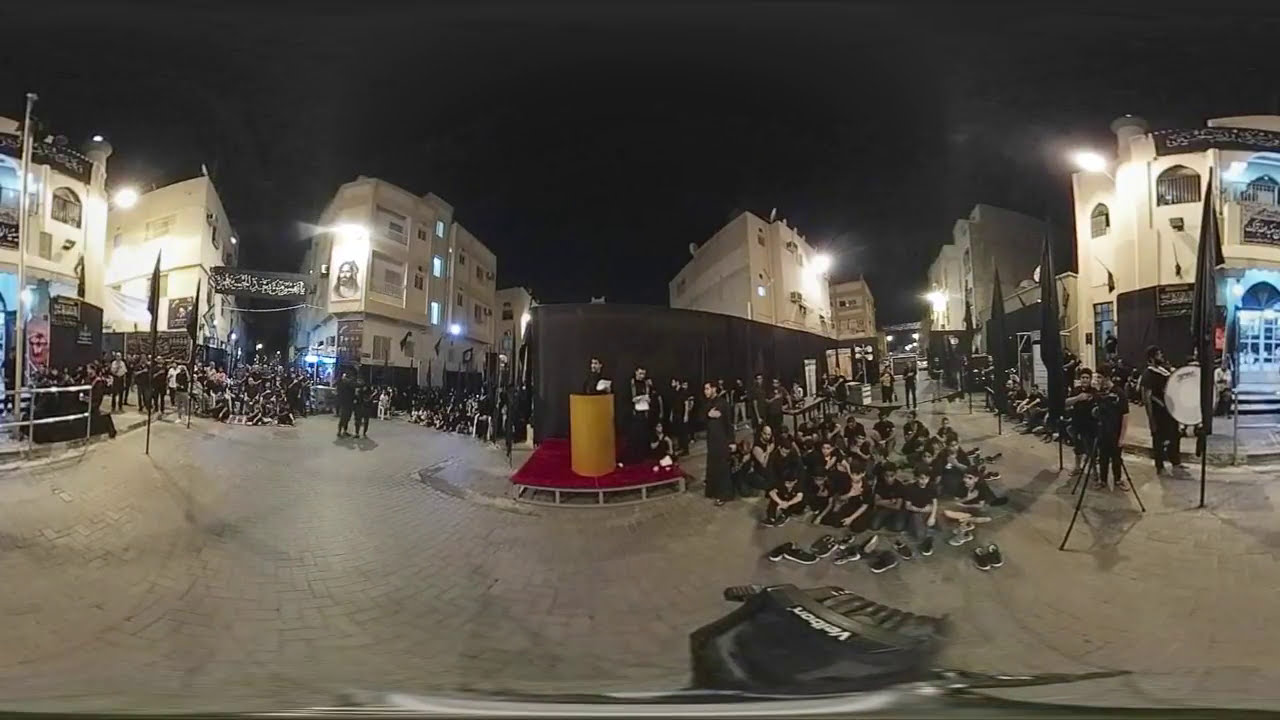The image captures a nighttime scene in a public square, characterized by cement-colored or white plaster buildings, possibly of Middle Eastern or hacienda-style architecture. The buildings are illuminated from within, contrasting the dark, black sky overhead. A large group of people, all dressed in black, are dispersed throughout the square—some standing, others seated on the ground, with many shoes visibly piled up. The scene suggests a significant event or gathering, marked by the presence of black banners atop the buildings, hinting at a festival, demonstration, or other organized event. Central to the image is a setup including a large pallet covered with a red cloth or padding and a yellow podium. Nearby, a large drum indicates that there may be a musical or ceremonial element to the gathering. The square, lit by the surrounding buildings, features a tile-like walking area where people are orderly clustered, and the overall atmosphere combines the vibrancy of an active public space with the solemnity of uniform attire and nighttime ambiance.